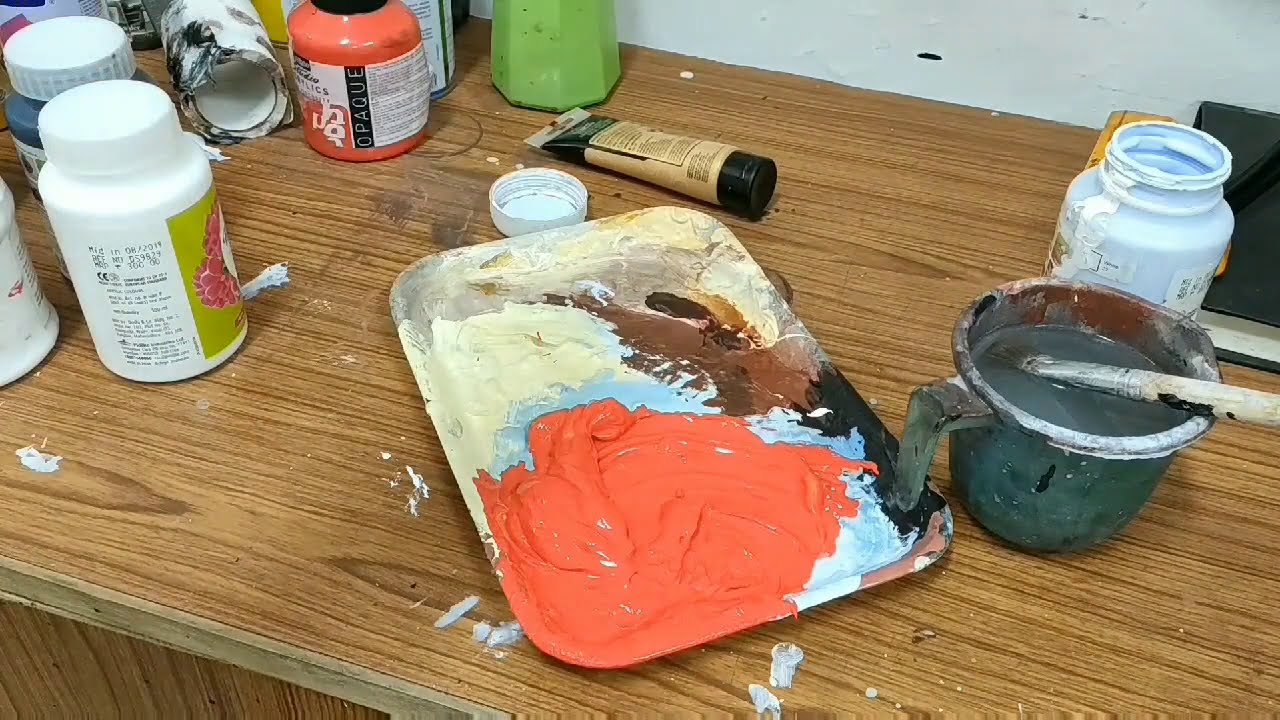In a cluttered workshop or garage, the scene showcases a messy wooden table sprawling from the upper left to the lower right of the image. At the center, a rectangular painting tray takes prominence, with various colors of paint splattered across it. Dominating the palette is a peach-orange hue, accompanied by splashes of light blue, dark green, brown, pale yellow, and white. Nearby, an assortment of paint bottles in shades of green, orange, blue, and white, possibly including a Mod Podge glue bottle, are strewn across the table. 

A small, murky measuring cup filled with dirty water and a paintbrush emerges as a focal point on the right-hand side of the tray. An open can of white paint, with its lid casually discarded behind, sits adjacent to the measuring cup. In the upper right corner of the frame, the gray cement flooring peeks through, adding to the disorganized ambiance. The only readable text within this chaotic array is on a paint bottle marked “opaque.” The scene vividly captures the vibrant, hectic energy of an active painting process.